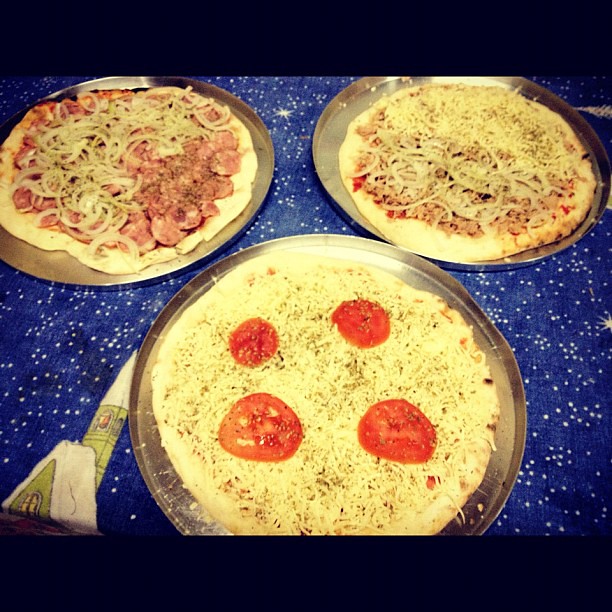The photograph showcases three unbaked pizzas on a blue table that is adorned with white star patterns, giving it a galaxy feel. The table also features a subtle design of a church steeple visible at the edge. The pizzas are presented on silver trays. The pizza at the bottom center features a simple arrangement of fresh cheese and four slices of tomato sparsely placed on top. In the upper left, there is a pizza loaded with toppings including onions, pepperoni or possibly sliced hot dogs, and cheese. The pizza in the upper right is also generously topped with onions and what appears to be ground beef or Italian sausage, with unmelted cheese scattered over it. The pizzas look ready to be baked with their raw toppings resting on pre-baked crusts.